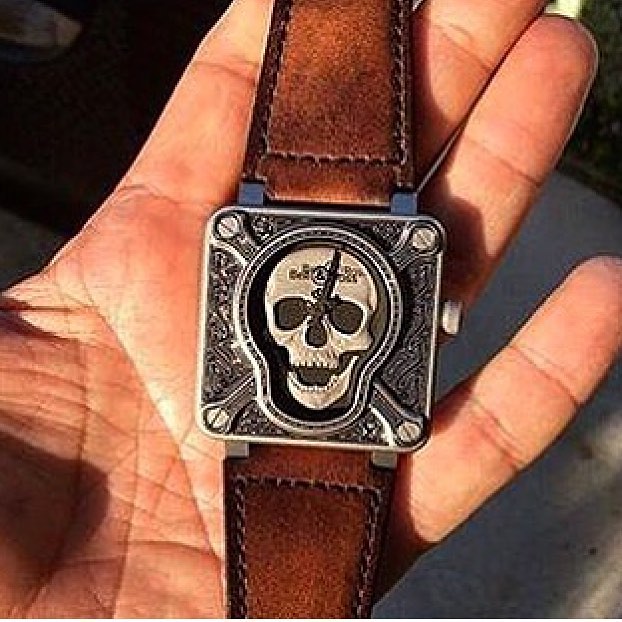The color photograph captures a close-up view of a person's hand, palm facing upwards, holding a distinctive square, flat object with rounded corners. This object features a menacing skull and crossbones design in black and gray, with the skull's mouth agape in an eerie expression. The background texture of the object includes intricate curvy black lines, adding to its intriguing appearance. The object rests atop a rich brown leather strap or band, meticulously detailed with brown stitching that accentuates its quality and craftsmanship.